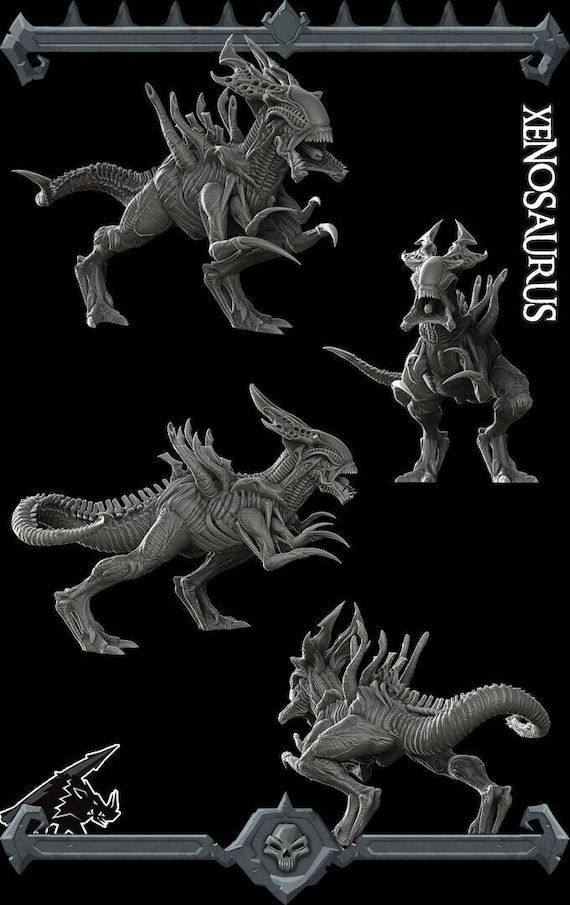This is an image, likely a digital rendering or a photograph of a poster, featuring a fictional creature called "Xenosaurus" highlighted in white text along the vertical right edge. The black background accentuates the gray, skeletal-like models of the creature displayed from various angles. In the top left corner, the side view showcases the Xenosaurus with a distinct crest on its head, tentacles, long talons, two legs, and a tail. Directly below, another view focuses on its open mouth, revealing sharp teeth. The middle left image gives a complete side profile, while the bottom right displays the rear view, emphasizing the tail and hind legs. A gray design borders the top and bottom of the image, with a skull logo centered at the bottom and sharp, tooth-like points at the top, enhancing the creature's menacing appearance.